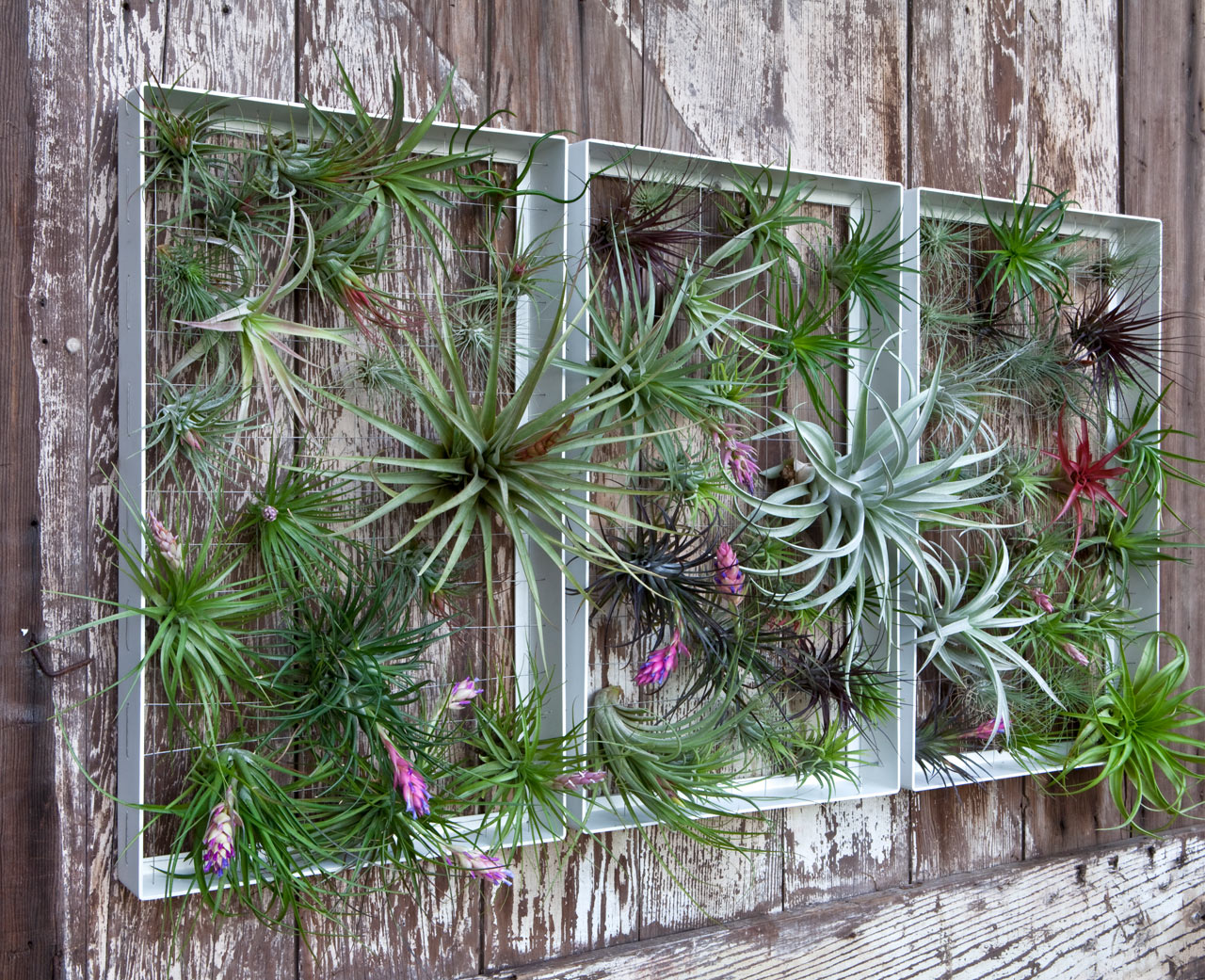In the image, there is a rustic wooden structure that resembles either an old barn door or a section of fencing. The wood appears weathered, as if it was once painted but now shows significant grain through the faded and chipped paint. This main wooden wall, which also includes wooden floorboards now partially overgrown with weeds, serves as the backdrop and the foundation for a unique display of air plants.

Mounted side-by-side on this wooden surface are three frames, devoid of bottoms and using the wood as their back. Inside each frame is a tight grid of wire supporting the air plants. These plants, which do not need soil, feature a variety of different species. The majority of the foliage showcases an array of green hues, with some plants having long, spiky leaves while others have more curved forms. Among the greenery, there are bursts of color: some plants bear pine cone-shaped pink flowers, and a striking red air plant is visible on the right. The scene presents a charming mixture of rustic wood and vibrant, spring-like plant life, emphasizing the natural beauty and diversity of the air plants on display.